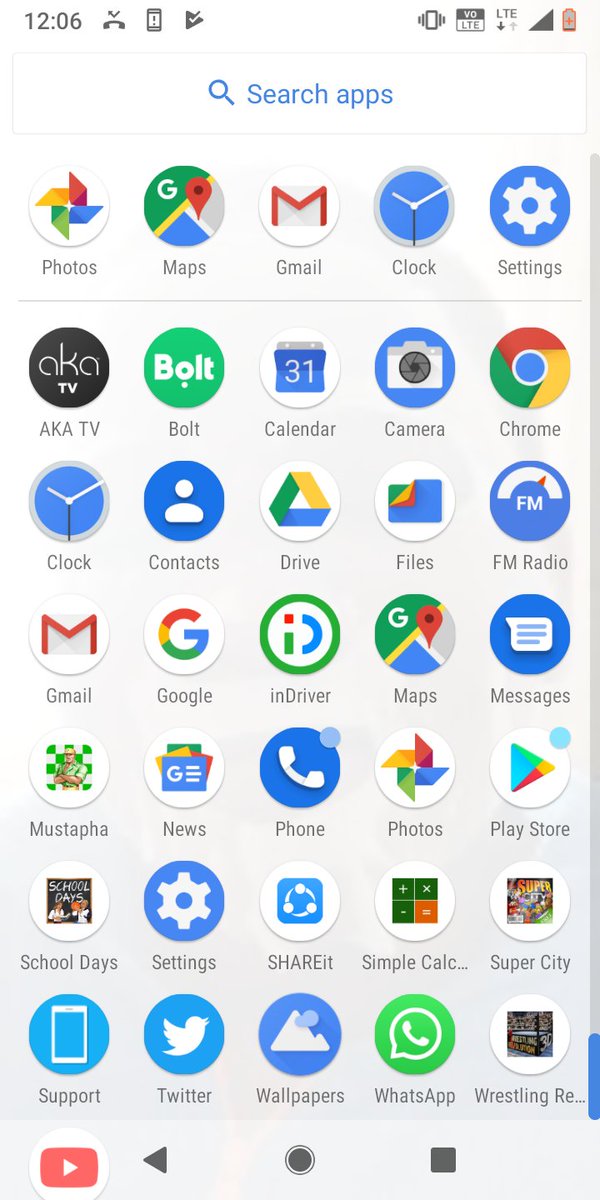The image showcases the home screen of an Android smartphone, prominently displaying the current time at 12:06. The status indicators at the top of the screen reveal a 4G LTE network connection and a battery level at 49%. A search bar labeled "Search apps" is positioned under the status indicators.

The screen is organized into rows of app icons, as follows:

1. **First Row**: Photos, Maps, Gmail, Clock, Settings
2. **Second Row**: AKA TV, Bolt, Calendar, Camera, Chrome
3. **Third Row**: Clock, Contacts, Drive, Files, FM Radio
4. **Fourth Row**: Gmail, Google, N-Driver, Google Maps, Messages
5. **Fifth Row**: Mustafa app, Google News, Phone, Google Photos, Play Store
6. **Sixth Row**: School Days, Settings, Share It, Simple Calc, Super City
7. **Seventh Row**: Support, Twitter, Wallpapers, Whatsapp, Wrestling Revolution

Additionally, a YouTube app icon is visible in the bottom left corner. At the very bottom of the screen, three typical Android navigation icons are present. Notably, the smartphone has a remaining battery life indicating that it may need charging soon.